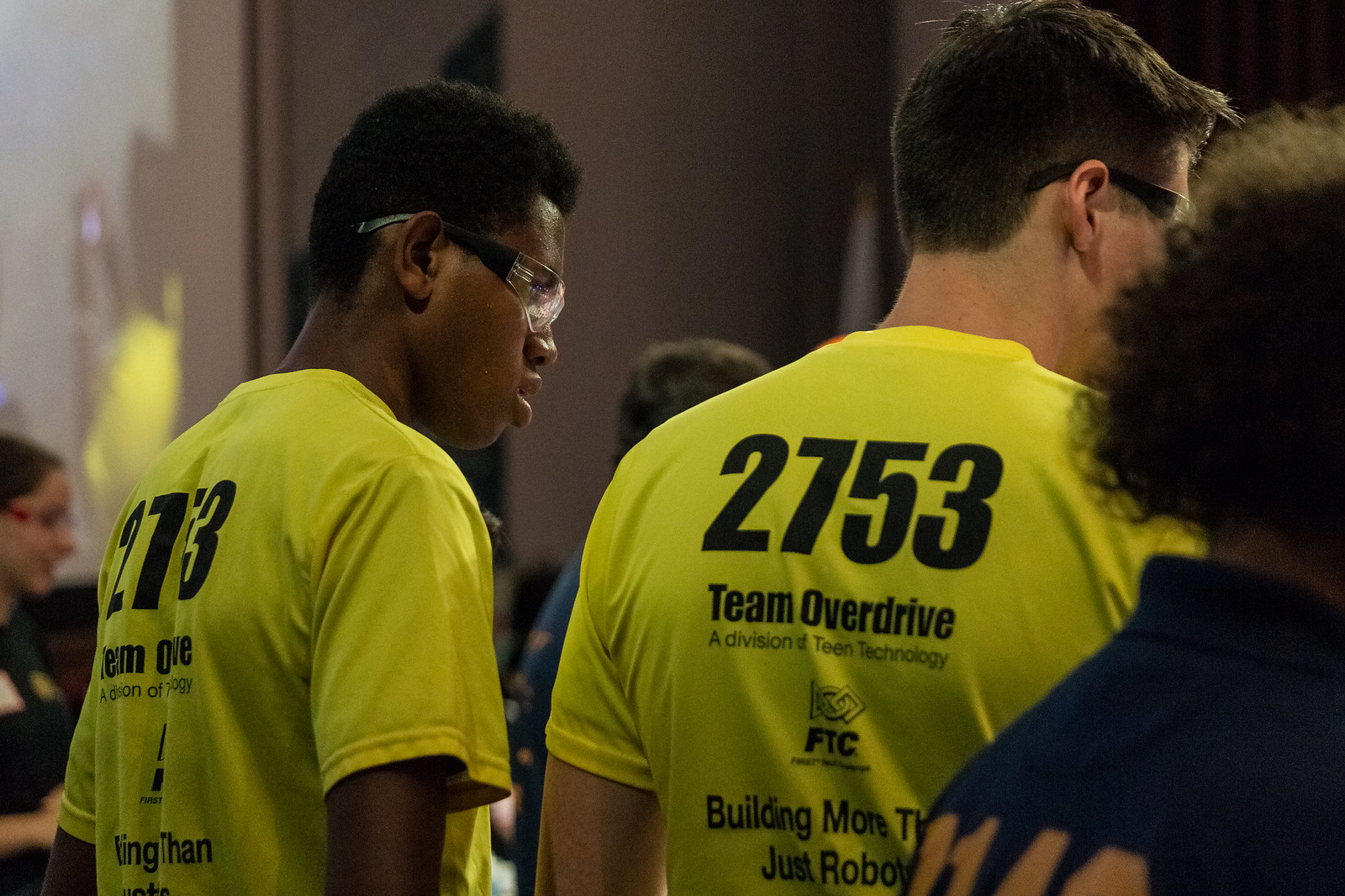In this indoor photograph, we see the backs of two individuals, centrally framed, both wearing bright yellow T-shirts with identical text that reads "2753 Team Overdrive, a division of D Team Technology." Below the text, there is a logo with the words "FTC" and "Building More Than Just Robots." The individual on the left, identifiable by his black skin and glasses, glances slightly to the left, revealing a partial side view of his face. The person on the right, who has white skin and also wears glasses, remains fully turned away from the camera. Both appear to be young, possibly teenagers, and have short hair. A third figure, whose gender is indiscernible, stands on the far right, wearing a dark jacket and showcasing very tight, curly black hair. The room is populated with other people, though they are blurred and less in focus, suggesting that the setting may be an active competition. The scene is suffused with colors of tan, gray, black, brown, lime green, red, and orange, adding vibrancy to the indoor environment.